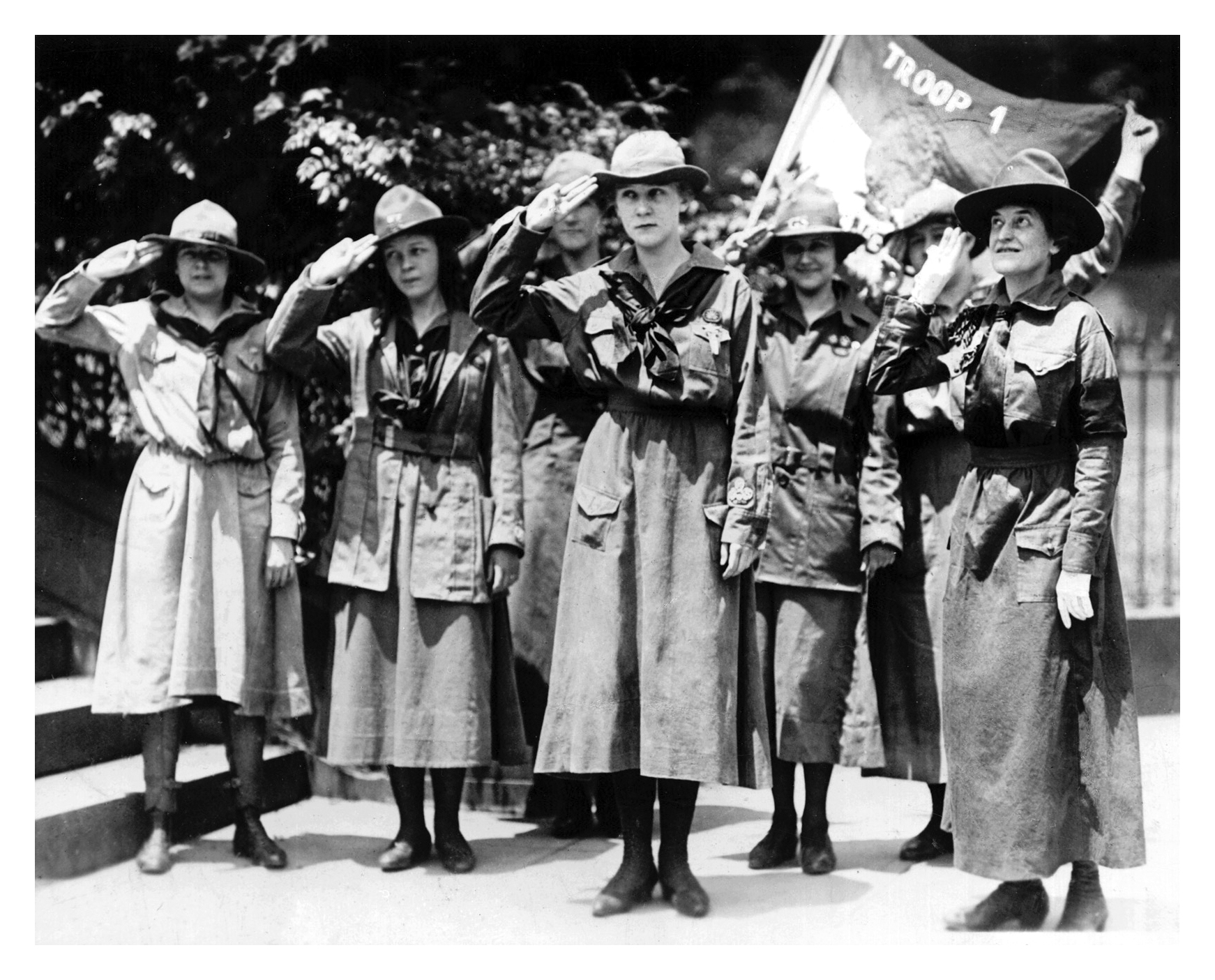This old black and white photograph shows a group of women, likely part of the Girl Scouts, dressed in scout uniforms. The uniforms consist of long skirts, tan blouses with long sleeves, wide-brimmed hats, scarves tied around their necks, and a combination of high heels and boots. They are all standing on a light-colored cement floor, saluting with a three-fingered gesture similar to the Boy Scout salute. In the upper right corner, a flag bearing the text "Troop One" is held by a woman at the back. The setting includes a stairway on the left and trees behind them, suggesting an outdoor location at the base of a building. The expressions on their faces vary; notably, a woman on the right side has an inquisitive look, as if questioning her presence there.